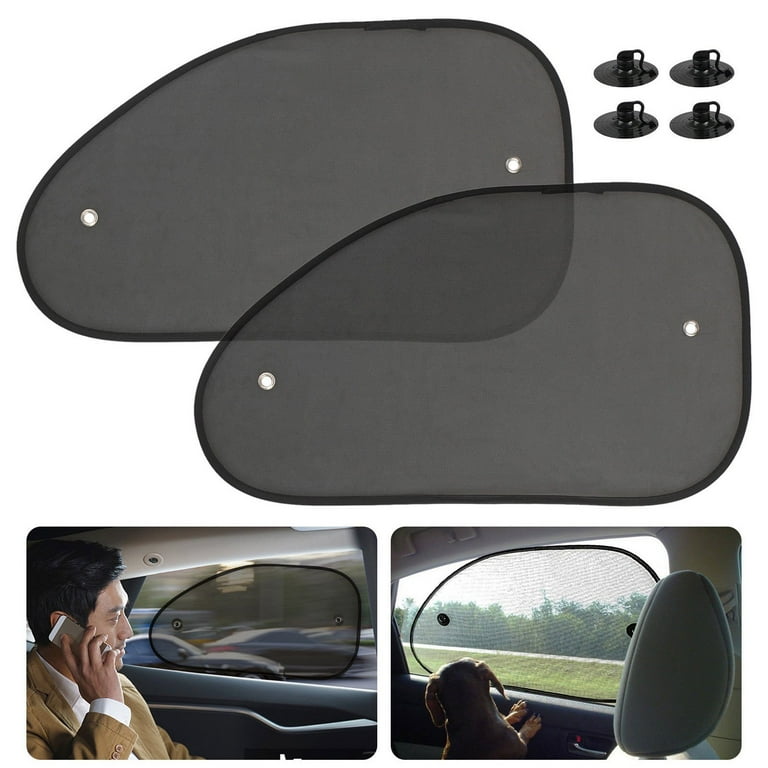The image showcases a set of black sunshield panels designed for car windows. The top section features two of these sun visors, shaped to fit the rear windows of a car, alongside four suction cup connectors used to secure them in place. The panels are shown stacked atop each other, emphasizing their functionality and ease of installation. 

Below, two practical application views demonstrate their effectiveness. In the first, a man wearing a brown jacket over a white shirt is seated in the car, engaged in a phone call, with the sunshield panel effectively blocking out harsh sunlight. The second image captures a small dog in the backseat, gazing out the window through the sun-filtering fabric, which prevents the animal from jumping or being tempted to jump out, and mitigates the glare. Both images highlight the panels' capability to reduce sunlight penetration, making the car interior safer and more comfortable. The bottom scenes emphasize real-life scenarios where the sunshields protect occupants from bright light and distractions. These might be promotional images from an advertisement showcasing the practical and protective uses of the product.